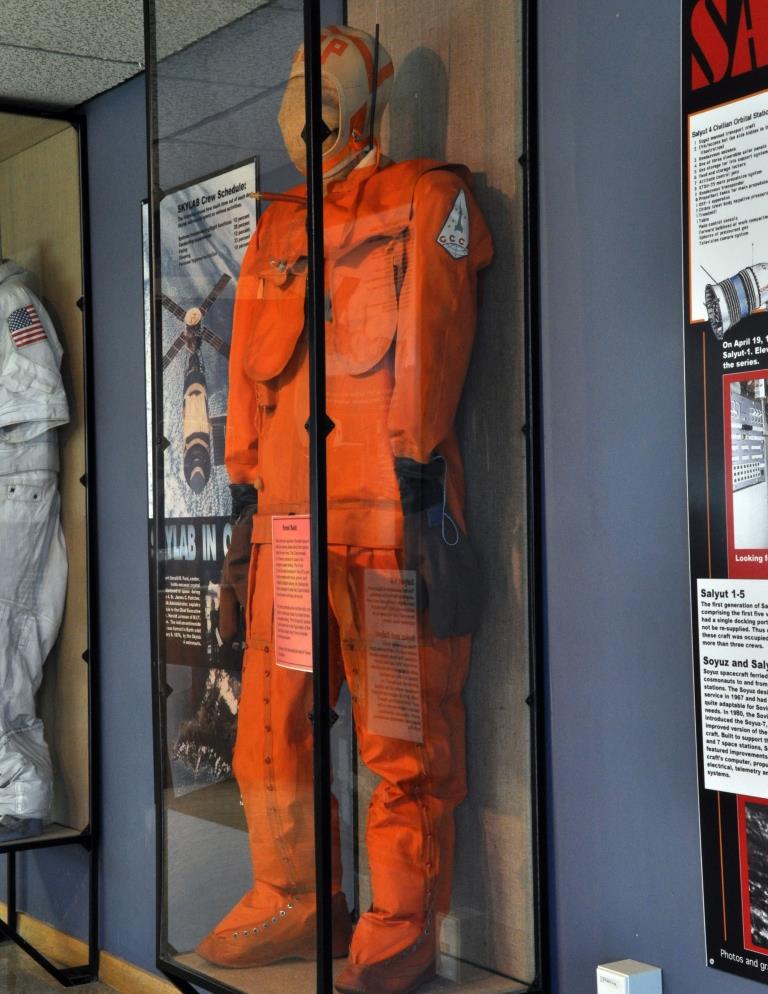The photograph was taken in a museum and prominently features a vividly orange, one-piece space or flight suit, likely a Russian cosmonaut uniform, displayed on a mannequin inside a clear glass case with a black frame and solid wood backdrop. The suit has integrated feet coverings and two large breast pockets. Distinctive details include a tan cap with partly visible letters ending in 'P' and a white sleeve patch near the shoulder resembling an arrowhead with 'CCC', potentially part of 'СССР' (USSR). To the right and left of the display, large posters provide informative text about the uniform's history and purpose. The adjacent exhibit partially visible showcases another suit adorned with a U.S. flag.